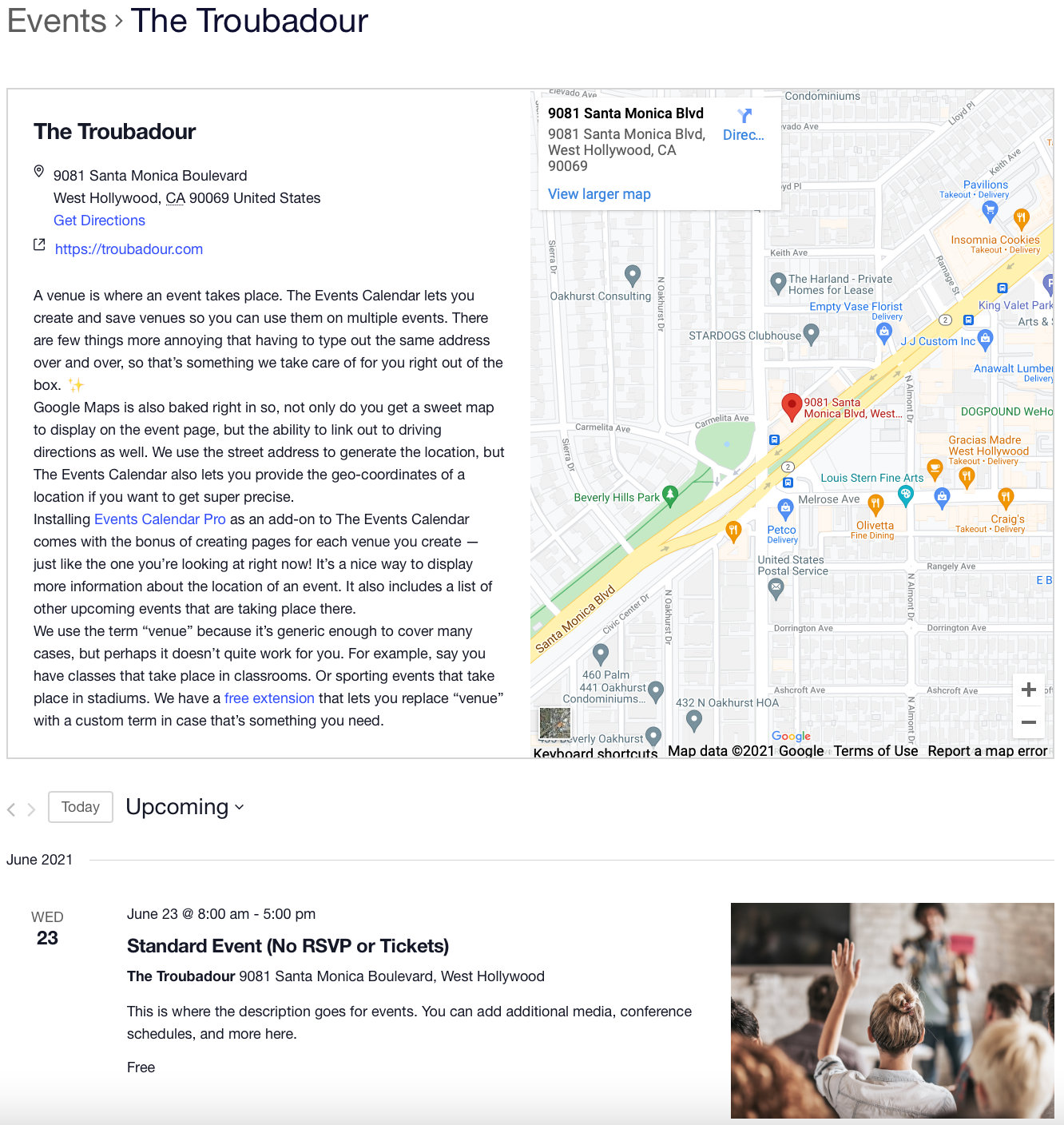**Detailed Caption:**

This image is a screenshot of a Google search result for "The Trobador," located at 9081 Santa Monica Boulevard, West Hollywood, California, 969 United States. The search result features a clickable link in blue text labeled "Get directions" and another link to the venue's website, "trobador.com." The text below provides an informative description, explaining that The Trobador is a venue for events, and detailing the functionality of the events calendar.

The calendar allows users to create and save venue details to avoid repetitive data entry, with Google Maps integration providing a convenient display of maps and directions. Users can input either the venue's street address or geo-coordinates for precision. The Events Calendar Pro add-on further enhances this by creating dedicated pages for each venue, displaying detailed information and hosting a list of upcoming events. 

To the right of the description is a map pinpointing the location at 9081 Santa Monica Boulevard and its surrounding area. Below the map, a schedule lists an upcoming event on Wednesday, June 23rd, 2021, from 8 a.m. to 5 p.m., described as a "standard event" with no RSVPs or tickets required.

Additionally, an image below the event description depicts people at an event, with someone raising their hand, illustrating a potential scene at The Trobador. This screenshot serves as a template for users wanting to create and manage event listings on the website or app, showcasing how the platform operates and how the formatted information would appear.